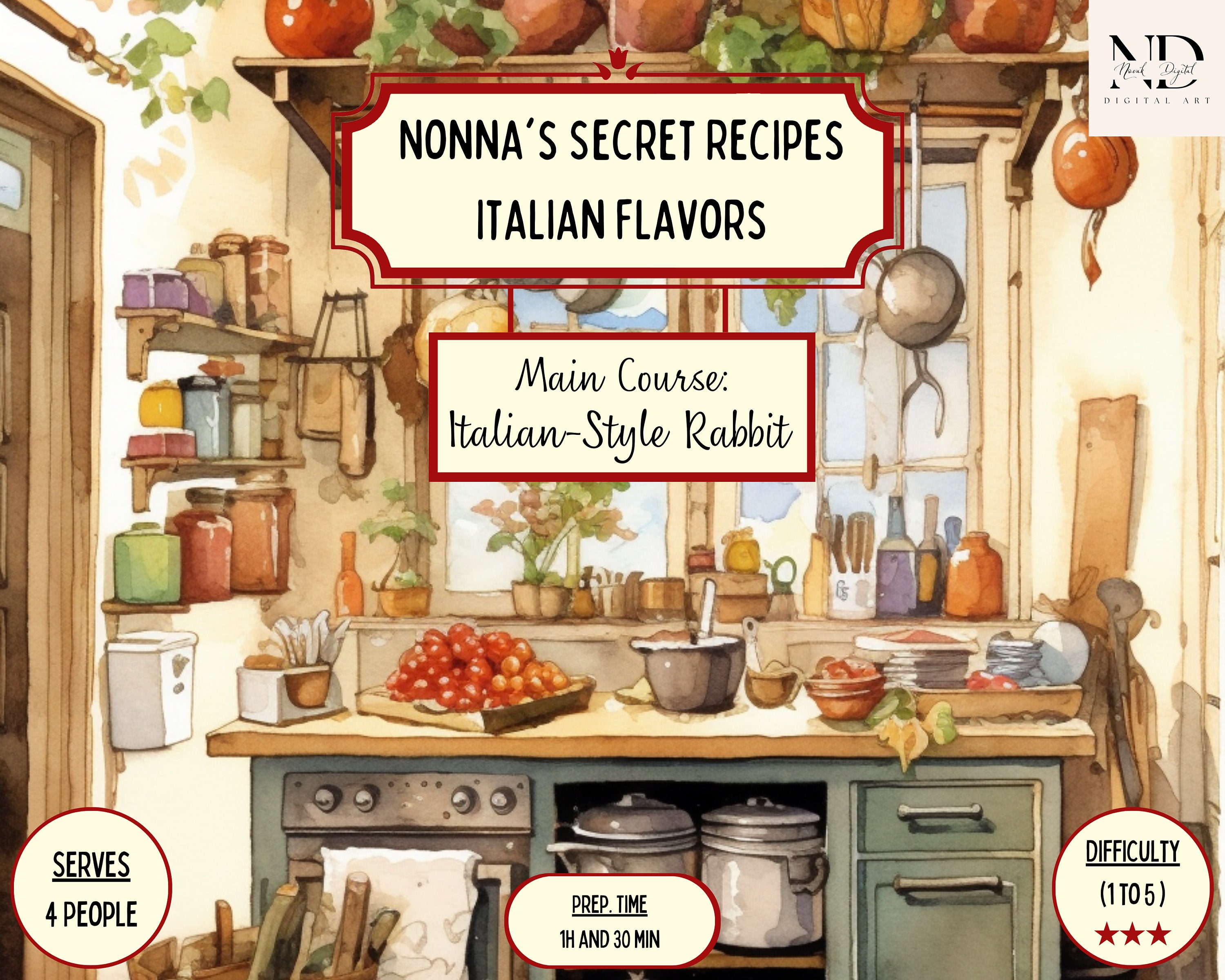This detailed image is the front cover of a cookbook, depicted in a watercolour style, showcasing a cozy kitchen setting. The background is a light yellow adorned with green leafy floral designs. A prominent title at the top reads "NONNA'S SECRET RECIPES" in all caps, with "Italian Flavours" below it, both encased in a milk-coloured platform with a red border. Below, a rectangular box features the main course, "Italian Style Rabbit," in a scripted font. The bottom right includes a circular platform indicating it serves four people. Prep time is noted as 1 hour and 30 minutes in a central oval platform, while difficulty is rated 1 to 5 with three red stars at the bottom left.

The kitchen scene is rich with details: shelves on the left house various baking jars in blue, tan, yellow, red, and green. The left side also features shelving containing flour, sugars, and baking items. The walls have a light yellow hue complemented by green leafy patterns. Pans hang from a top shelf, and a window with green trees outside frames the backdrop. On the countertop, a heap of tomatoes sits on a brown wooden cutting board. A blue bowl filled with something white and several other bowls, including an orange one, add to the kitchen’s clutter. A central silver stove is flanked by a small silver cabinet with drawers, and a cubby holding large stock pots. The foreground showcases additional kitchenware, a pot with a ladle, and a tray of assorted items.

A logo reading "ND Digital Arts" is located in the top right corner, tying in the artistic theme of this cookbook cover. The meticulous details of kitchen utensils, food items, and the picturesque setting evoke a homely and appetizing atmosphere perfect for a collection of cherished Italian recipes.